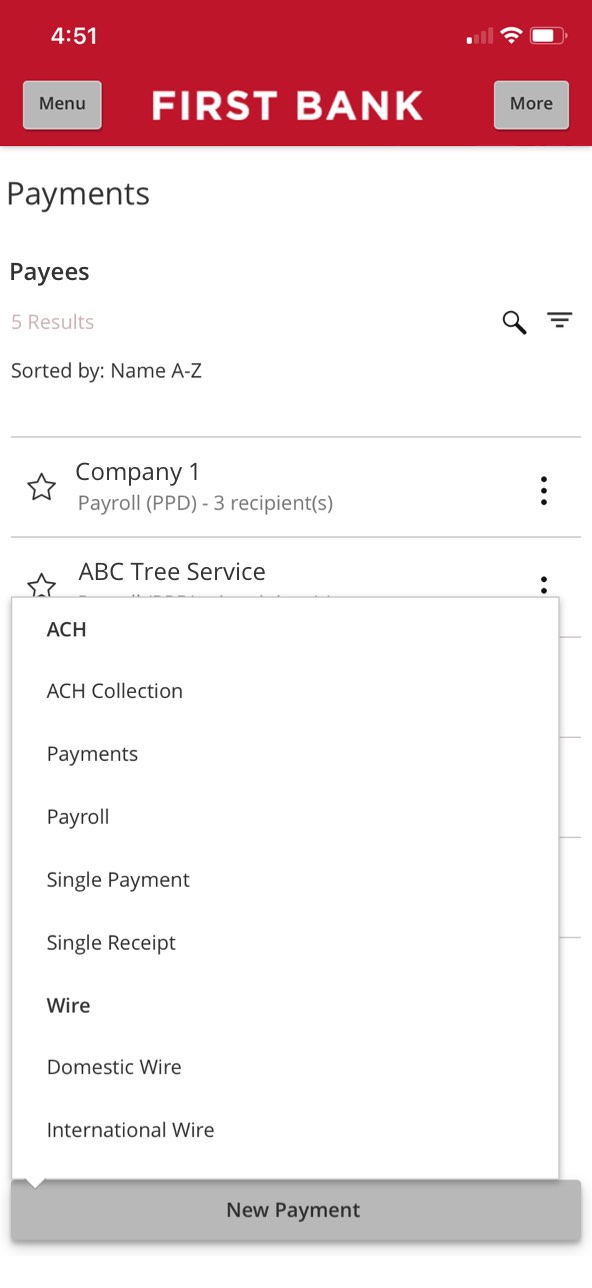**Descriptive Caption:**

Screenshot of First Bank's online banking interface displayed on a mobile phone. The top portion of the screen features the First Bank logo in white font on a deep red background. Flanking the logo are two grey buttons labeled "Menu" and "More" in black text. Above this section, the phone's status bar is visible, showing the battery level, Wi-Fi, and signal strength, as well as the current time of 4:51.

The main body of the screen presents a clean, minimalist online banking interface dominated by a white background with black text. The top heading reads "Payments, Payees," followed by a list of five payees sorted by name. Below this, a search bar allows users to find specific entries. The first listed payee is labeled "Company 1, Payroll, PPD, 3 Recipients."

A highlighted menu on the right side includes options such as ACH, ACH Collection, Payments, Payroll, Single Payment, Wire, Domestic Wire, and International Wire. At the bottom of the screen, a grey button with black text invites users to "Make a New Payment." The overall look is straightforward and functional, designed to facilitate easy navigation and efficient financial management.